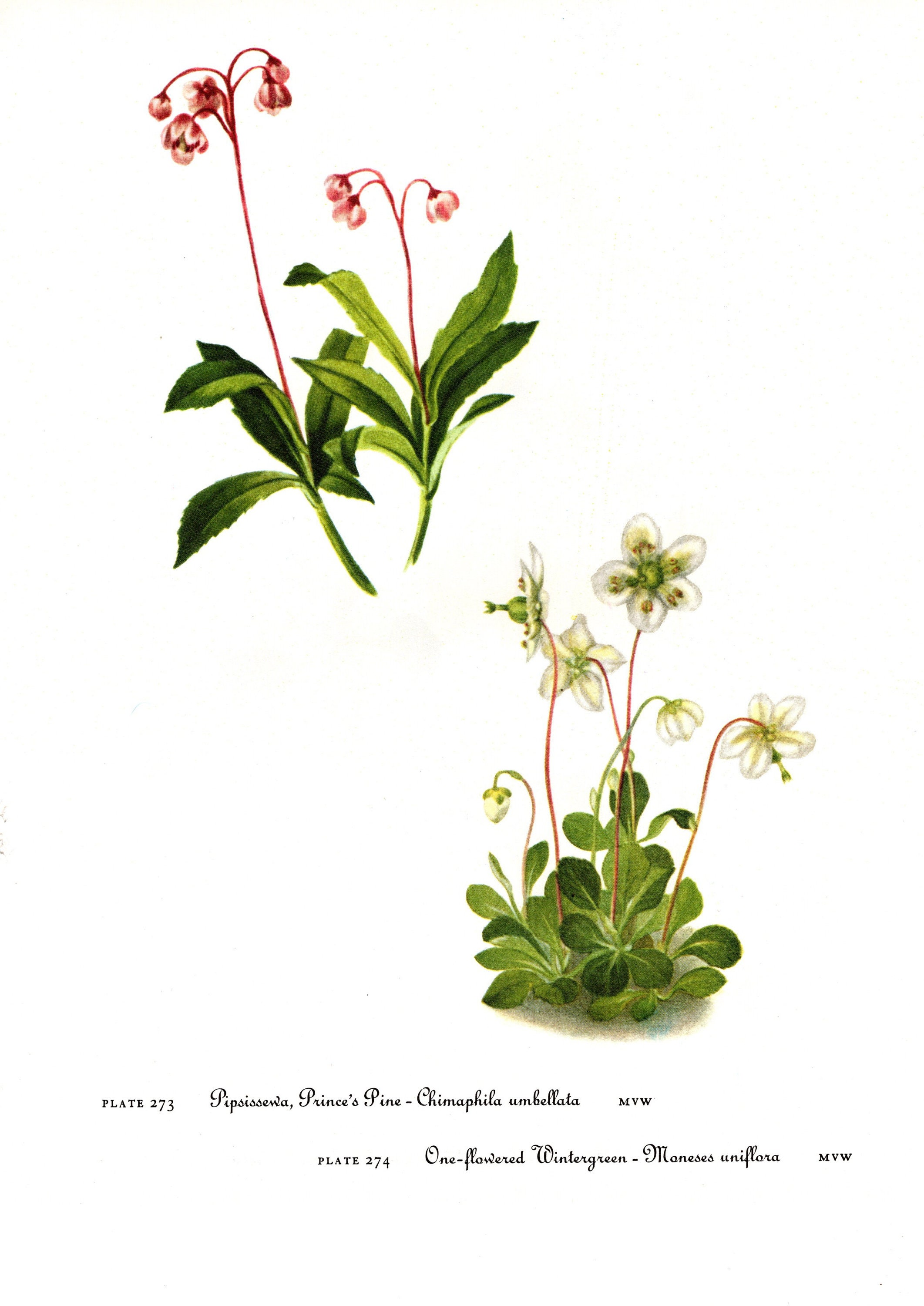This image features two detailed botanical illustrations of flowering plants, set against a blank white background. In the upper left-hand corner, labeled Plate 273, is an illustration of a plant identified as "princess pine, chymphyllia, umbrella" (though the exact wording is unclear), showcasing long, pointed green leaves at its base, and red flowers with yellow centers that droop downward from long, red vines. The plant in the bottom right-hand corner, labeled Plate 274, appears to be "one-flowered wintergreen, [some word starting with M] uniflor, MVW" (though again, the exact wording is difficult to read). This plant features shorter, more rounded, oval leaves at the base, with reddish-pink stems that give rise to white flowers with green interiors and small yellow segments. The illustrations have a realistic feel, almost as if from an old flower guidebook, and are accompanied by small cursive text that is challenging to decipher.